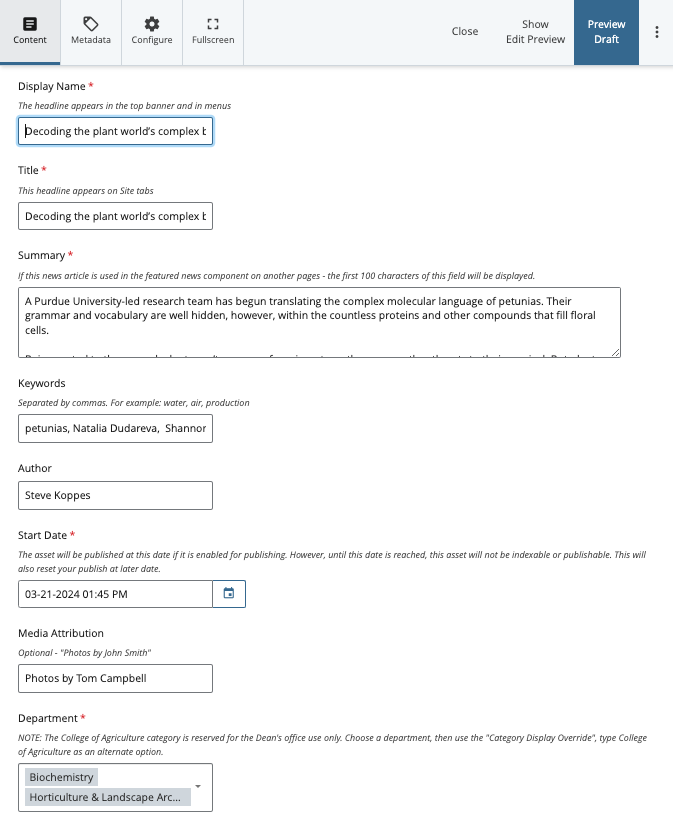***Decoding the Plant World's Complex Language: Unveiling Petunias' Molecular Grammar***

A Purdue University-led research team has embarked on the ambitious task of translating the complex molecular language of petunias. Despite the intricacies, their vocabulary and grammar are embedded within countless proteins and other compounds that populate floral cells. Led by Natalia Dudareva and Chang-Ho Chang, and reported by Steve Kopp, this groundbreaking study delves deep into understanding the subtle yet sophisticated signals that control plant physiology and interactions. Scheduled for a digital release on March 21, 2024, at 1:45 PM, this research could redefine our approach to horticulture and biochemistry. Photos capturing the essence of the study are attributed to John Smith and Tom Campbell. This detailed exploration, categorized under 'Biochemistry, Horticulture, and Landscape Art' in Purdue's College of Agriculture, promises to shed light on how decoding plant molecular communication can lead to advancements in agricultural practices and our comprehension of plant biology overall. 

Keywords: petunias, molecular language, floral cells, proteins, Purdue University, Natalia Dudareva, Chang-Ho Chang.